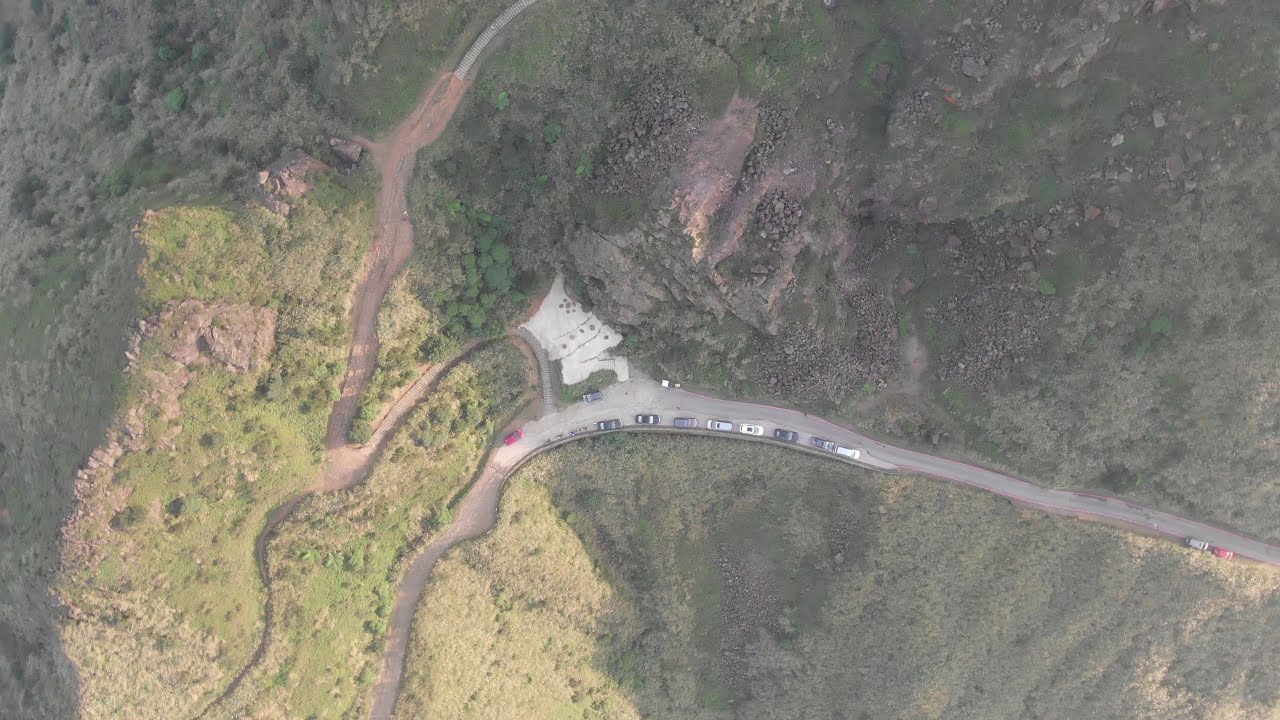This image is a detailed aerial shot of a mountainous area captured from a high altitude, displaying a landscape orientation. At the center of the photograph, a road, initially asphalt, traverses from the bottom left corner towards the center and then veers off to the right. This road transitions into a dirt path towards the left side of the image, leading into rougher terrain. Alongside the road, there are about eight cars parked, indicating a possible trailhead or turnout area with a white sandy surface, suggesting a starting point for hiking trails that meander through the terrain.

The right side of the image is characterized by lush greenery, while the left side becomes more yellowish-brown due to the increasing prominence of dirt and rocky outcroppings. The photograph also captures a small white structure with a driveway, standing out amidst the natural setting. The overall color palette includes green, yellow, brown, black, white, and red, reflecting the diverse elements within the scene. Taken from a straight-down perspective, this drone photograph vividly represents the realism of a rural, outdoor mountainous environment during the day, showcasing both natural beauty and functional elements like roads and trails.